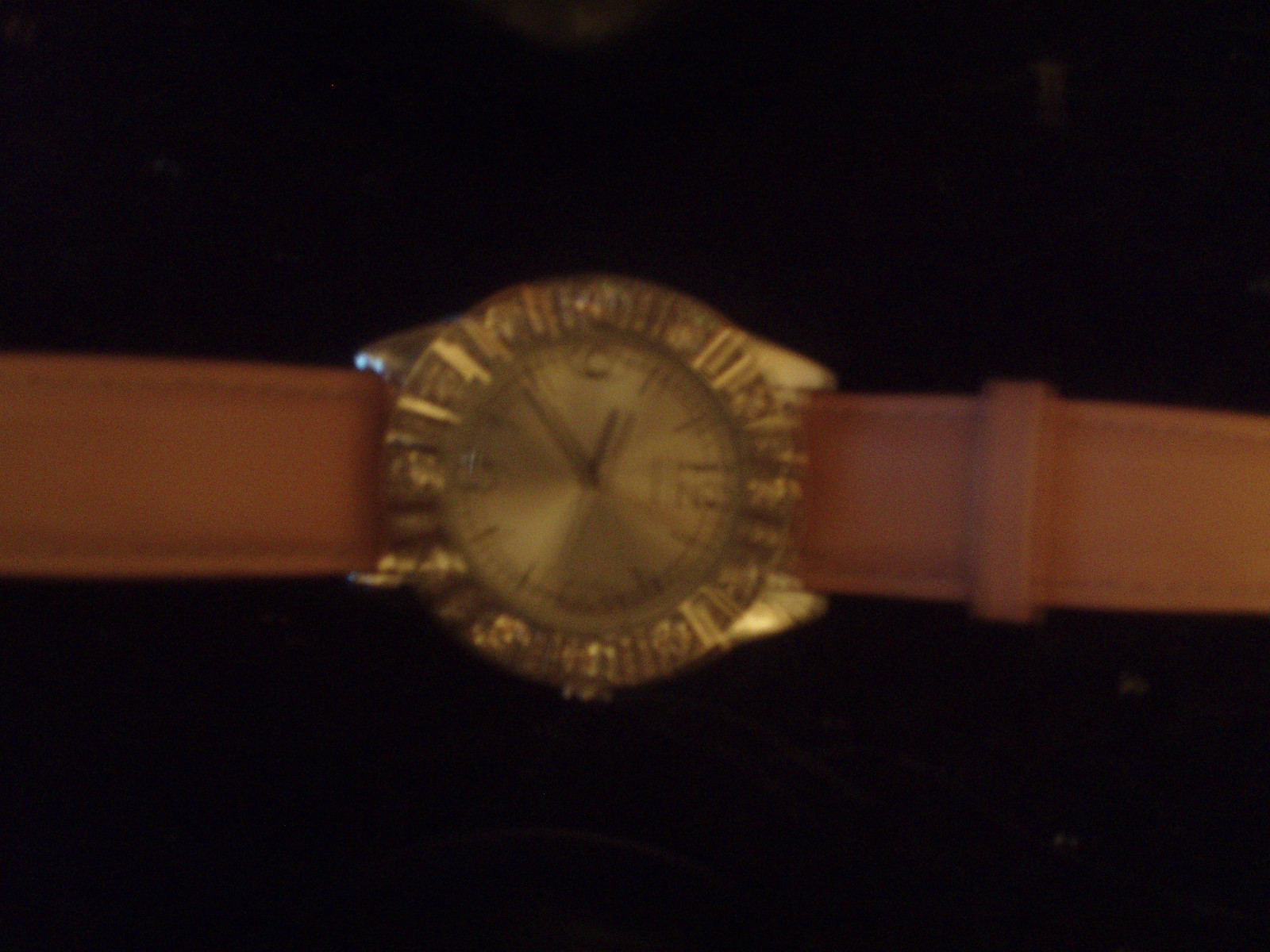The image depicts a women's wristwatch laying horizontally at an angle on a black background with some tan and brownish-purple abstract marks. Despite the blurriness, the details of the watch can be seen: it has a light brown leather strap, a round silver watch face lined with diamonds, and black hands indicating the time is 9:40. Large numbers mark the 12, 3, 6, and 9 positions on the face, adding an old-school charm to the otherwise elegant piece.